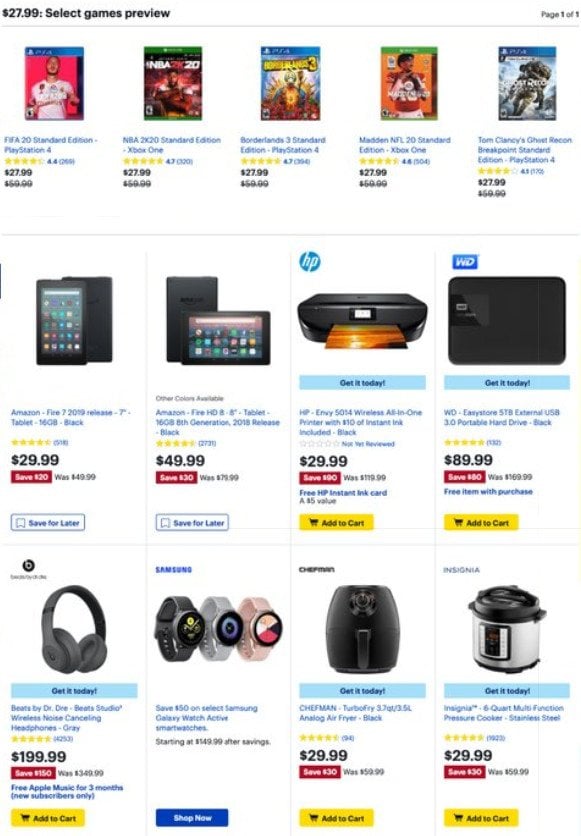This is a web page from a website that sells a variety of products, including games and electronics. At the top of the page, against a black background, the price $27.99 is prominently displayed. Below that, there is a selection of game previews. Featured here are five games: 'FWA 20 Standard Edition' for PlayStation 4, 'NBA 2K20 Standard Edition' for Xbox One, 'Borderlands 3 Standard Edition' for PlayStation 4, and 'Madden NFL 20' for PlayStation 4.

Further down, the page showcases an Amazon tablet, followed by another tablet to the right. Next to these is a wireless all-in-one printer. To the right of the printer, there is a portable hard drive. Below these products, the page features headphones, smartwatches, an air fryer, and a pressure cooker. Each item comes with customer ratings and an option to add them to your cart. Overall, this section presents a diverse array of products including games, tablets, smartwatches, printers, external hard drives, pressure cookers, and air fryers available for purchase.